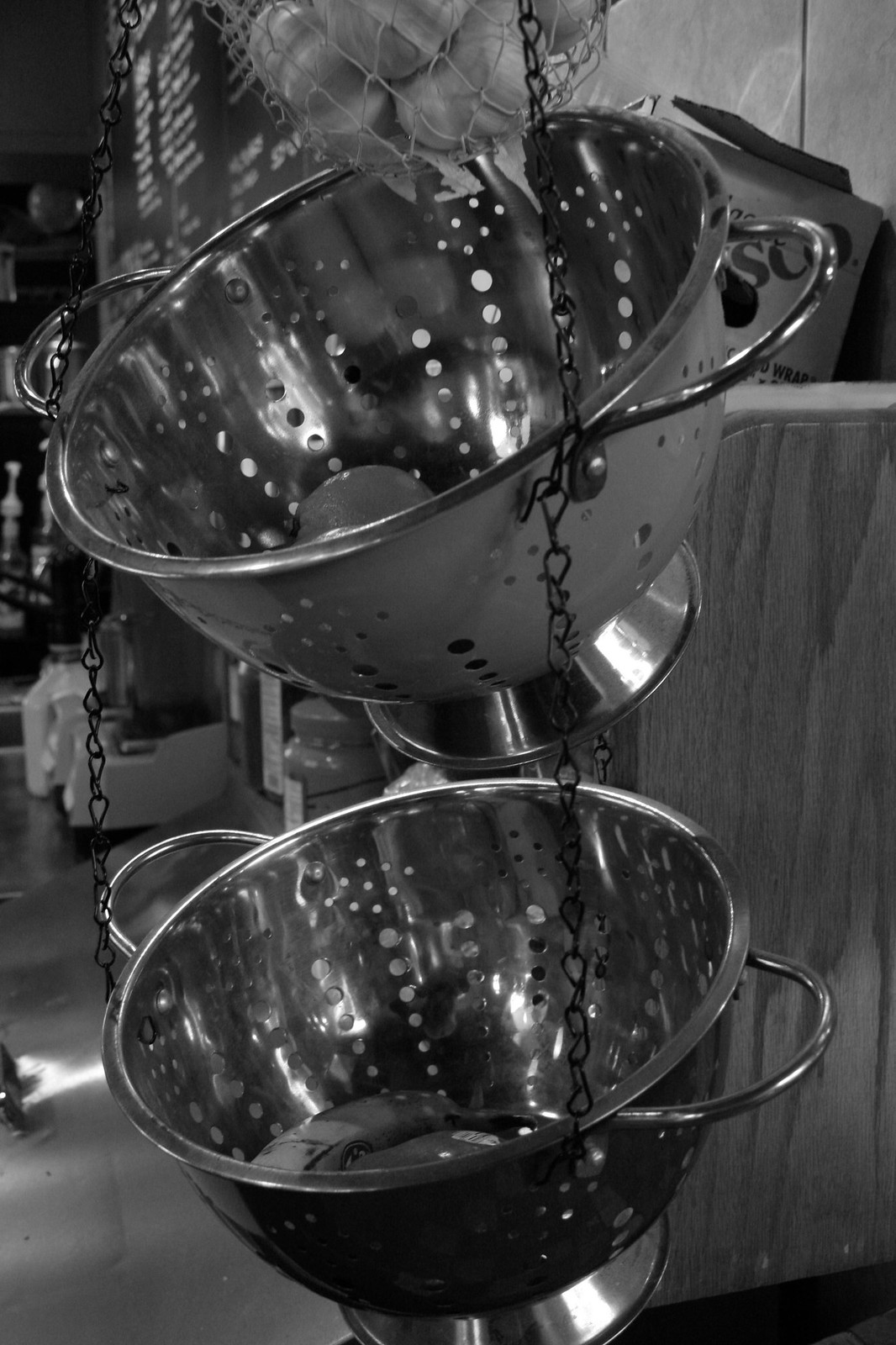The black and white photograph, taken indoors in portrait mode, features two metal colanders suspended from the ceiling by black chains. The colanders, each with rounded metal handles and a flared base, are tilted slightly, revealing their interiors. They resemble strainers with numerous holes. The top colander contains a white mesh bag filled with garlic, some of which hangs loosely from the bottom. The bottom colander appears to hold bananas. Behind these colanders stands a wooden shelf, partially obscured and shaded in various grays due to the grayscale photography. Atop this shelf sits a cardboard box with the letters 'SCO' visible. To the side, there is a dark menu board adorned with indistinct white text, and some very high shelving is apparent in the darker upper corner of the image. The right side of the frame is dominated by a wooden wall, suggesting a possible restaurant-style kitchen setting.